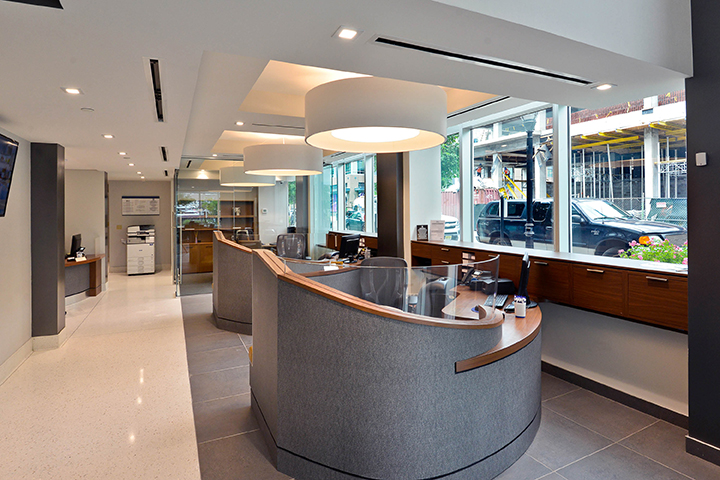The photograph captures the interior of a modern, white-themed reception area, possibly within a hotel lobby or office space, characterized by its contemporary decor and an abundance of natural light. Central to the image are round, gray-coated reception desks, each resembling its own small, circular island equipped with a gray office chair, a slightly outdated black computer monitor, keyboard, and phone system. These desks are complemented by clear glass barriers, adding to the sleek, modern aesthetic. The floor contrasts in a pristine white marble, while the ceiling features numerous large, circular lights. To the right, a series of expansive windows reveal parts of parked vehicles and a building under construction, with hints of tree leaves visible through the glass. In the background to the left, a photocopy machine is noticeable next to another reception area with a similar black computer monitor, underscoring the workspace function of the area. An additional element is a TV tucked into the left corner, further contributing to the office's multifunctional setup.